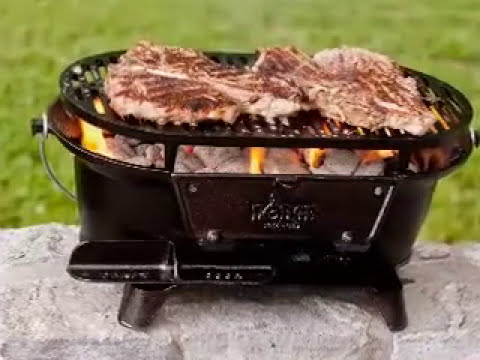The image depicts a close-up of a small, black, oval-shaped Lodge brand mini charcoal grill, reminiscent of an old-fashioned tub with its raised four black peg legs. The grill is perched on a fairly flat, gray stone surface, with blurred green grass visible in the background. The grill has a rectangular plaque on its front, with a name that starts with an "L," though the exact text is unreadable. The black grate on the grill, raised about half an inch, holds two large T-bone steaks that have been flipped to cook the other side. Below the grate, white-hot charcoal pieces emit flames that almost touch the steaks, indicating an active cooking process. The image quality is moderate, lacking high-resolution detail, and it focuses closely on the grill and the food, with no additional people, objects, or text present in the photograph.